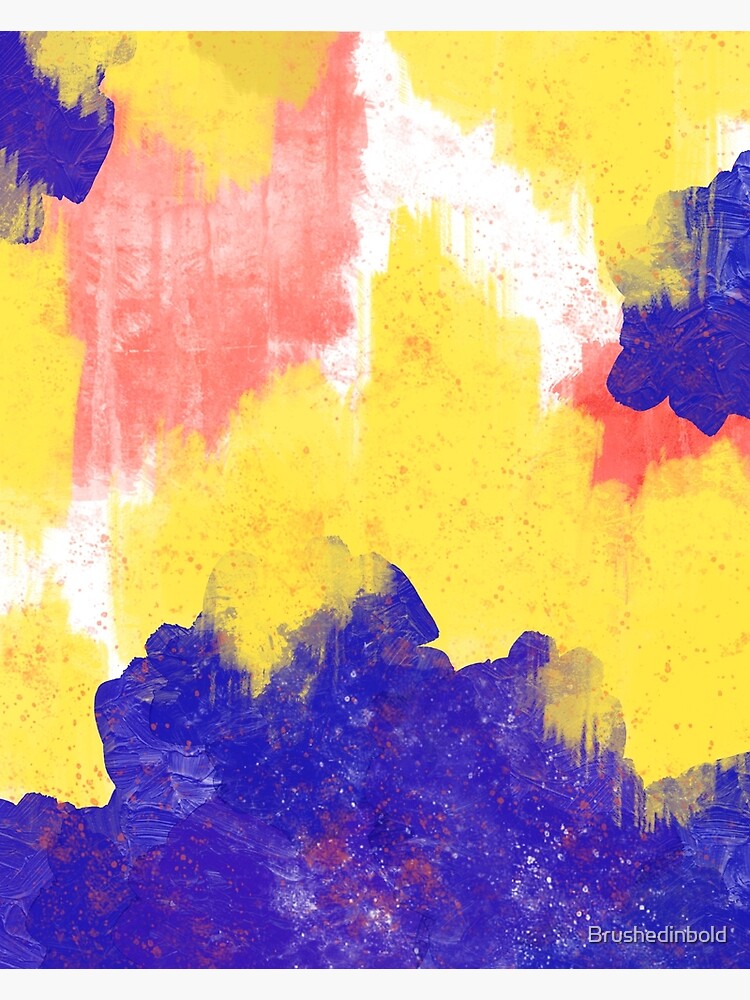This image is a close-up photograph of an abstract painting, characterized by bold brushstrokes and a texture suggesting oil or acrylic paint. Dominated by large blocks of yellow, purple, and peach colors, the composition creates a striking visual contrast. Flecks of peachish-pink and white are scattered across the yellow and purple areas in a droplet pattern, adding depth and movement. The top middle features white spots, while the left-hand side, two-thirds from the top, also shows a section of white with similar droplets. Blue tinted cloud-like forms appear on the top and bottom parts of the painting, intermingling with streaks of light reddish color. The bottom right corner bears a small, detailed script reading "brushed in bold," subtly integrated into the artwork. Despite its seemingly random and abstract nature, the painting exhibits noticeable brushstrokes and a textured canvas surface, offering a visually rich and intricate experience.